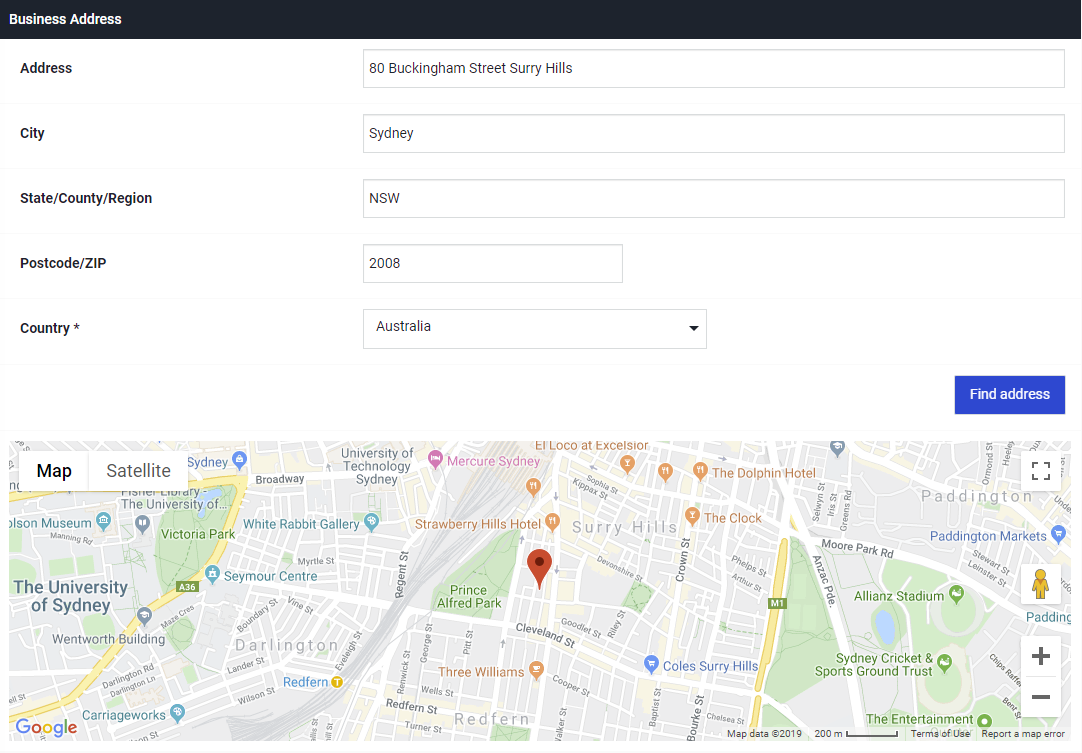The image features a black border at the top, with the white text "Business Address" located in the upper left-hand corner. Directly below this title, the form presents several labeled fields. 

The first field is labeled "Address," with an address box to its right, filled in with "80 Buckingham Street, Surry Hills" in black text. The next field is labeled "City," with an adjacent box containing "Sydney.” Following this, there is a field labeled "State - County - Region" flanked by the entry "NSW," likely denoting New South Wales.

The subsequent field is "Postcode - ZIP," populated with the code "2008." Below this, the "Country" field, marked with an asterisk to signify a required field, displays the chosen country as "Australia."

In the bottom right-hand corner, there is a blue button with white text that reads "Find Address." Beneath this button, a map resembling a Google Street View Map of Australia is displayed, with distinct elements identifying it as such. 

In the map's bottom left-hand corner, the Google logo is visible. The top left corner of the map section features two buttons: "Map" (bolded) and "Satellite." The top right corner includes a large icon, while below it on the right side, there is the "human" icon for entering Street View mode. Additionally, plus and minus symbols for zooming in and out are also positioned here.

Several notable points are labeled on the map, including "University of Sydney," "Sydney Cricket and Sports Ground Trust," "Allianz Stadium," "Paddington," "Paddington Market," and "Surry Hills." The location icon is centered, slightly to the left of "Surry Hills."